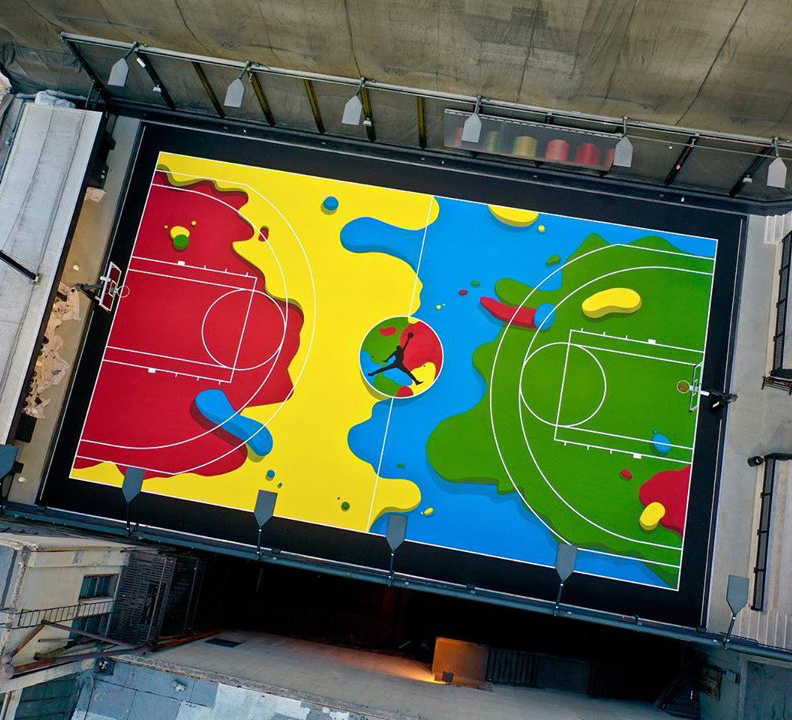The image depicts a vibrant basketball court, probably situated on the rooftop of a city building. The court stands out due to its vividly painted floor, which features an intricate blend of colors. The court is divided into sections: one end is splashed with red, the opposite end with green, and the middle areas showcase yellow and blue segments, evenly spread from left to right. At the very center of the court is a circular design, which incorporates all these colors—green, yellow, blue, and red—and showcases a silhouette of a basketball player holding a ball, possibly in a jumping pose.

The view is from an elevated angle, looking down onto the court, which is bordered by black fencing. Surrounding the court, on the upper side of the image, there is a gray wall, while the lower part reveals an urban setting with buildings interspersed by open spaces. Basketball hoops are present at both ends of the court, and the entire scene is cast with a dynamic, almost mural-like quality that suggests it may be a tribute or homage to basketball culture, possibly even Michael Jordan. The court's bright flooring and overall artistic design make it a striking focal point amid the surrounding cityscape.